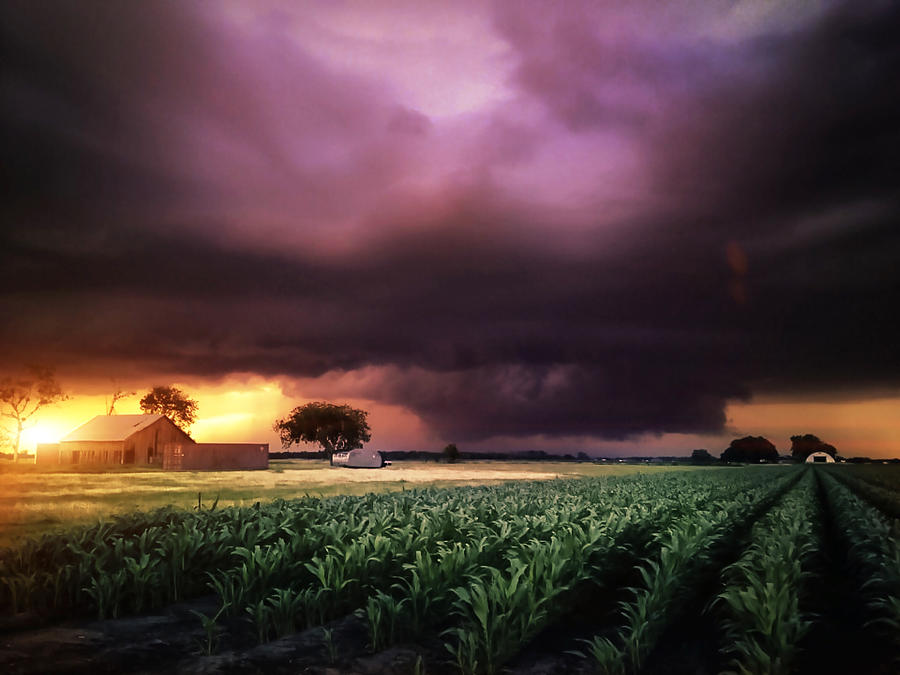In this realistic photograph of a farm at dusk, dark, menacing clouds dominate the sky, giving an impression of impending stormy weather, perhaps even hinting at a tornado. The sun, nearly set, casts a faint, fleeting light across the scene. On the left side, a barn or farmhouse is visible, surrounded by three tall trees. Adjacent to it, there's a vintage metal-style camper trailer. In the near foreground and stretching towards the horizon, rows of either corn or soybean crops are beginning to grow, their evenly spaced green lines creating orderly patterns in the field. A white, dome-shaped garage-style building stands on the right. Further into the distance, a silo and additional trees can be seen, contributing to the farm's expansive and open layout. The entire landscape is enveloped in a moody, grayish-black sky, enhancing the sense of an approaching storm.